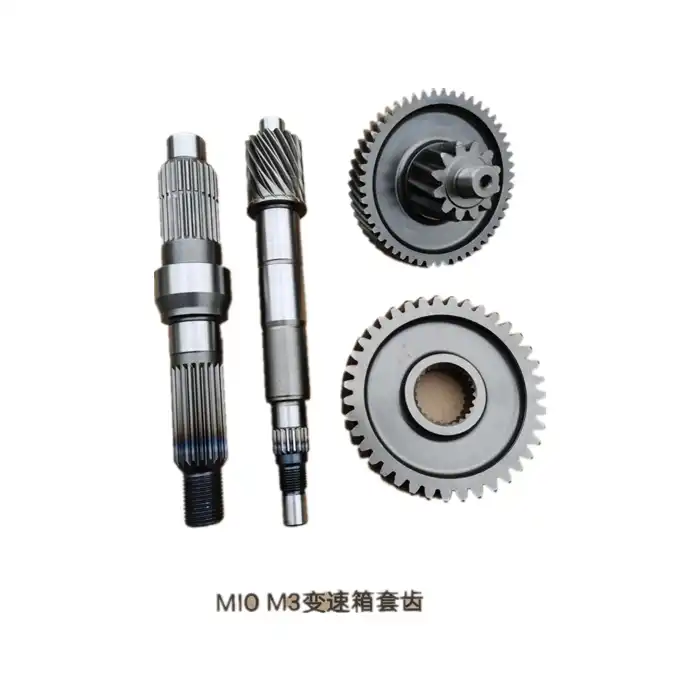The image showcases four metal machine parts set against a solid white background. On the left, there are two long vertical cylindrical pieces, each featuring alternating textures of smooth and grooved sections. The far-left piece has a smooth segment at the top followed by a grooved area, a bolt-like feature in the middle, and finishes with additional grooved sections and threaded rings at the bottom. Next to it, the other vertical piece alternates between smooth and grooved textures, including three or four smooth segments interspersed with two grooved areas. On the right side, there are two circular gears with jagged edges, one positioned above the other. The top gear has a nut in the center, while the bottom gear has an empty hole in its middle. The longer cylindrical pieces appear to be designed to fit into the gears, facilitating connection or assembly. Below these items, some text is visible, reading "M10" and "M8," followed by a series of characters in either Japanese or Chinese. The entire setup consists solely of these metal components, displaying a uniform metallic sheen.